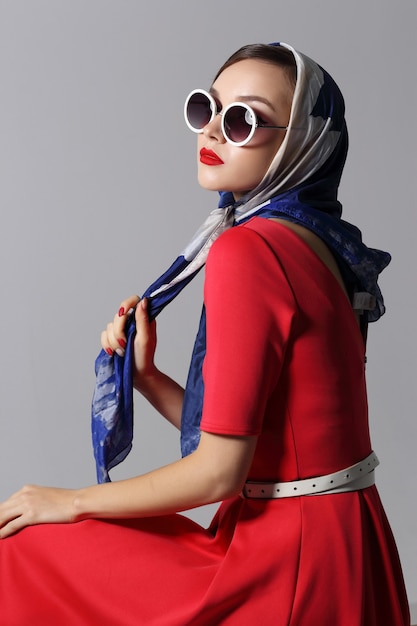This photograph captures a young woman, who resembles a model, positioned right of center against a light gray background. Her slender body is turned to the left, while her head, crowned with dark hair, is twisted slightly back toward the viewer, offering a glimpse of both her left profile and front. She is adorned in a vibrant red dress with sleeves ending just above the elbow, cinched at the waist by a thin white belt. Elegantly draped over her head and neck is a blue and white scarf, part of which falls over her back and loops in front. The woman wears large, round sunglasses with white rims that accentuate her red lipstick. Her hands are poised gracefully; her left arm rests on her bent knee, signaling a sitting posture, while her right hand clutches one end of the headscarf. Her red-painted fingernails add a touch of sophistication to her overall look.